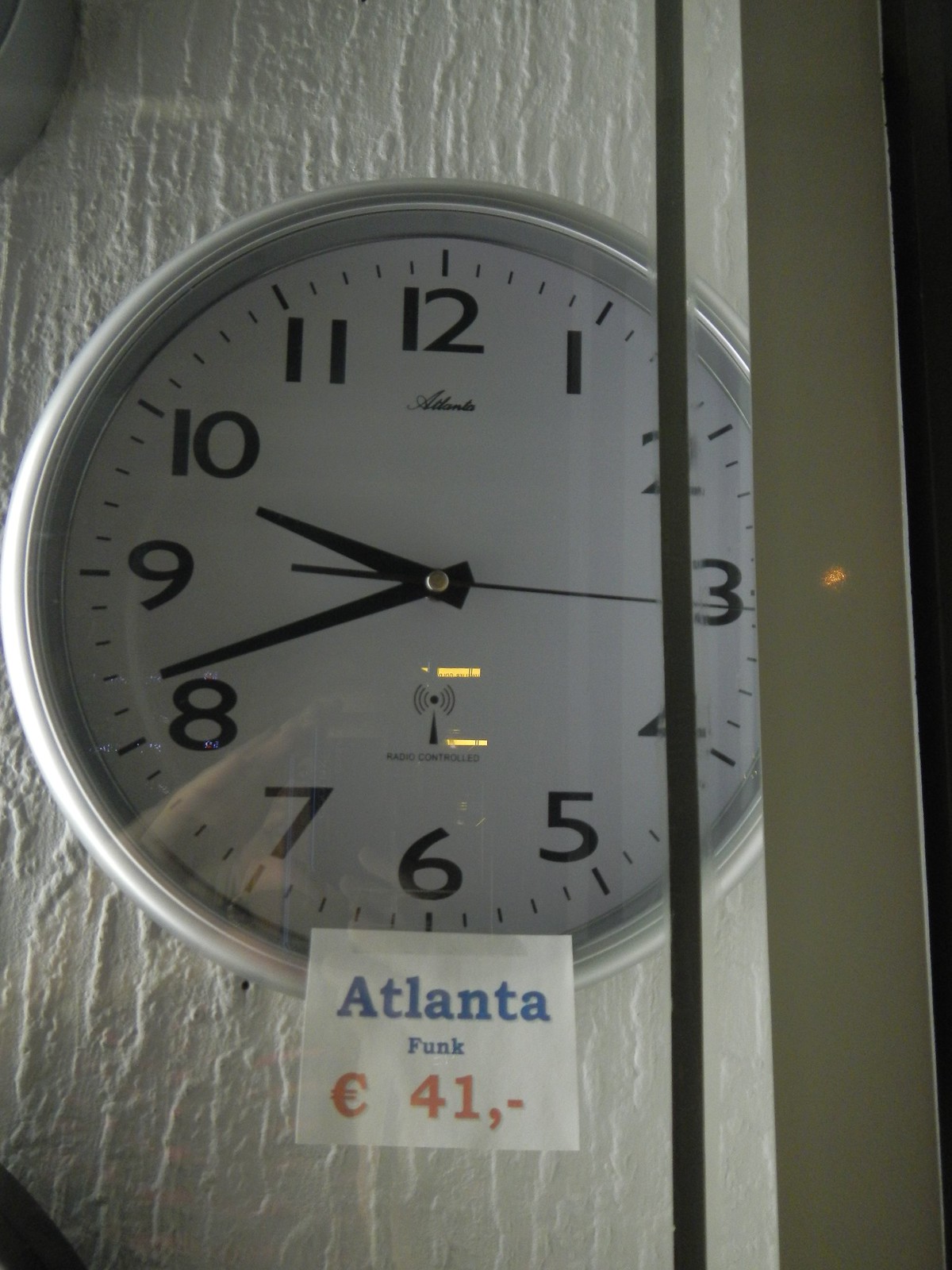In the center of the image, we see a circular clock hanging on a wooden wall, visible through what appears to be a glass door with a white border. The wooden wall is white with several vertical markings. The clock itself features black numbers arranged in their typical positions, with the 12 at the top, the 3 on the right, the 6 at the bottom, and the 9 on the left. The shorthand points closer to the 10, and the long hand is nearer to the 8, with a seconds dial at the 3. The clock face is light gray with a silver circular frame. Below the clock, there appears to be white styrofoam. At the bottom middle of the glass door, there is a white square sticker with the text "Atlanta Funk" in blue and "41 cents" in orange. To the right of the door, a gray bar is visible against a slight black background.